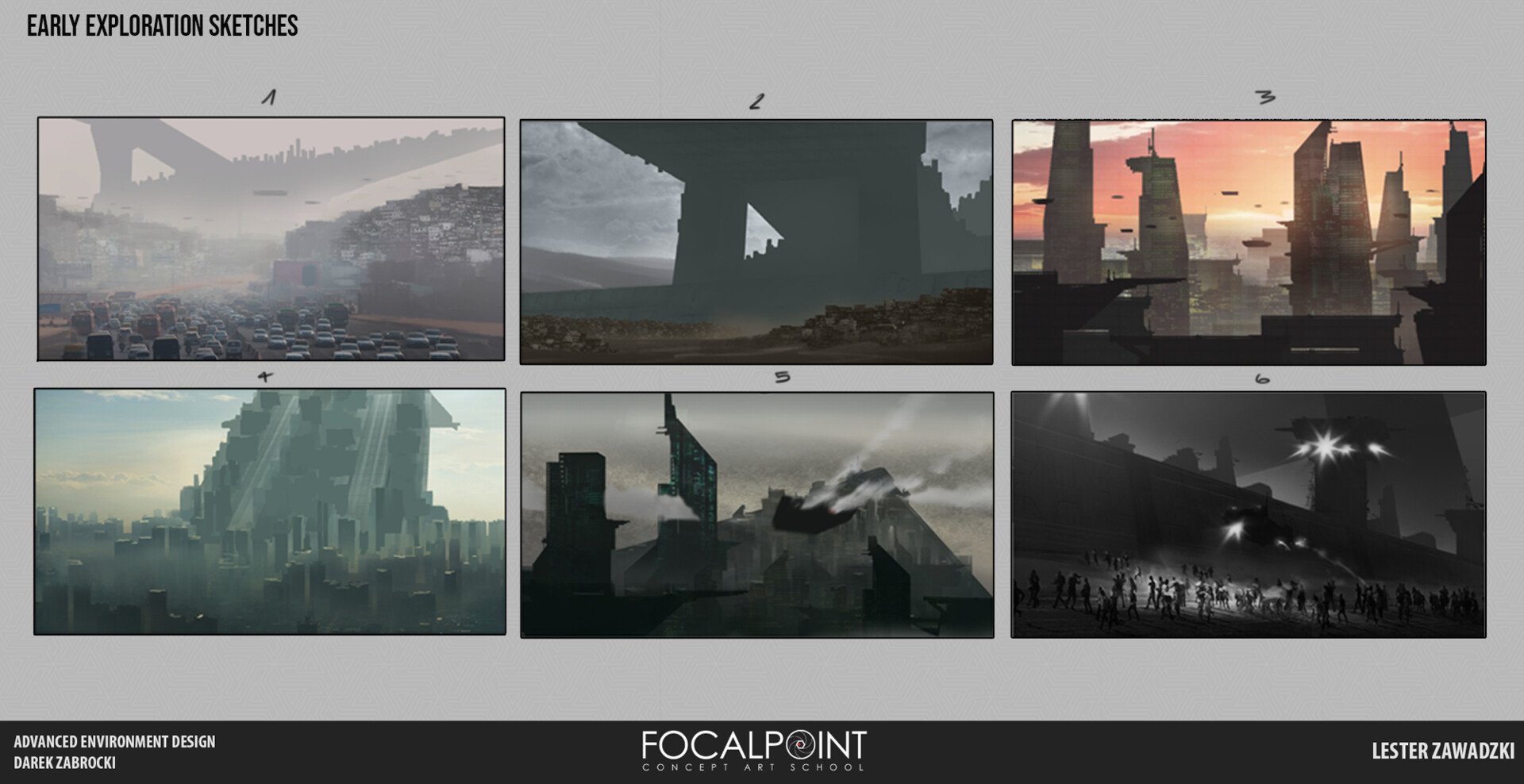The image is a collection of six detailed, grayscale environmental concept sketches, displayed in a 3x2 grid format on a gray background. Each sketch, measuring the same size, showcases various post-apocalyptic or dystopian cityscape scenes, suggesting scenarios such as a spaceship landing, decaying urban environments, and imposing structures. A notable detail includes the upper-right sketch featuring a sunrise backdrop that adds a touch of color to the primarily monochromatic palette. Text elements frame the artwork, providing context and attribution: "Early Exploration Sketches" at the top, "Advanced Environment Design" on the left, "Focal Point Concept Art School" in the center, and names "Derek Zabrocki" and "Lester Zawinski" on the right. The overall feel conveys intricate, imaginative settings likely intended for a movie or video game project.